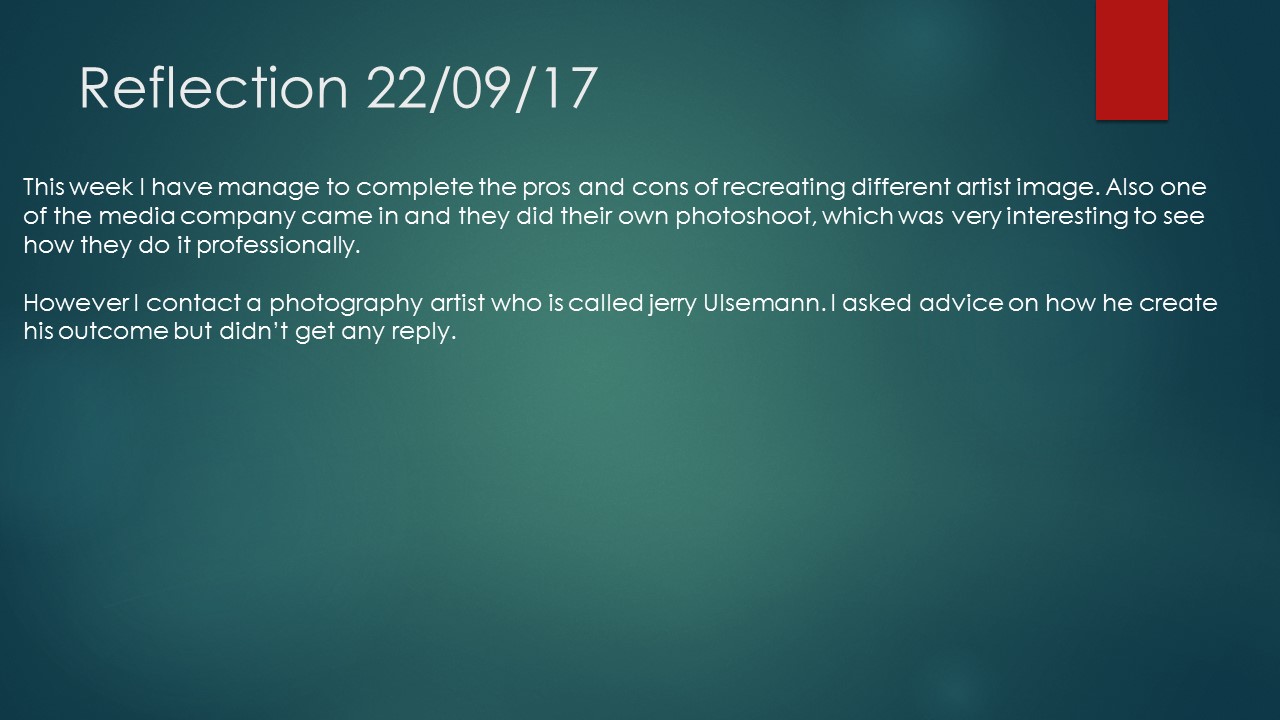The image resembles a PowerPoint slide or informational presentation with a color-rich background transitioning from dark teal green to a lighter sea green towards the center. A short red banner extends down from the top right corner. In the upper left, large white text reads "Reflection 22-09-17." Below it, two paragraphs of smaller, left-aligned white text describe recent experiences: "This week I have managed to complete the pros and cons of recreating different artists' images. Also, one of the media companies came in for their own photo shoot, which was very interesting to see done professionally. However, I contacted a photography artist named Jerry Olseman for advice on his creative process, but unfortunately, did not receive a reply." The overall style blends graphic design with typography, creating a visually engaging yet informative layout.